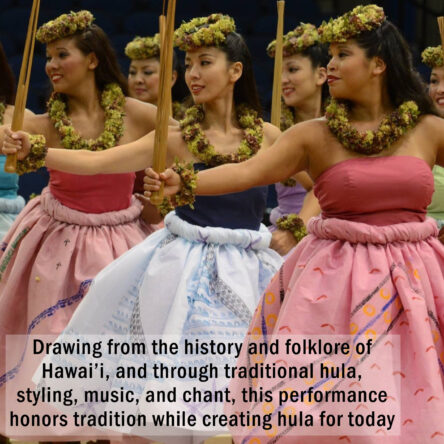The image depicts six women adorned in vibrant hula attire, positioned in two rows. The three women in the front row are more prominent. From left to right, the woman on the far left is slightly further back and wears a red top with a pink skirt. The middle woman is attired in a black top paired with a blue skirt, while the one on the far right mirrors the first with a red top and pink skirt. All the women have yellow floral wreaths on their heads, along with yellow and purple leis around their necks and wrists. They hold sticks in their hands and are facing slightly to the left and forward. The heads of three women in the back row are visible between the bodies of the front row. Below the group is a transparent white rectangle featuring four lines of black text that reads: "Drawing from the history and folklore of Hawaii and through traditional hula, styling music and chant, this performance honors tradition while creating hula for today."